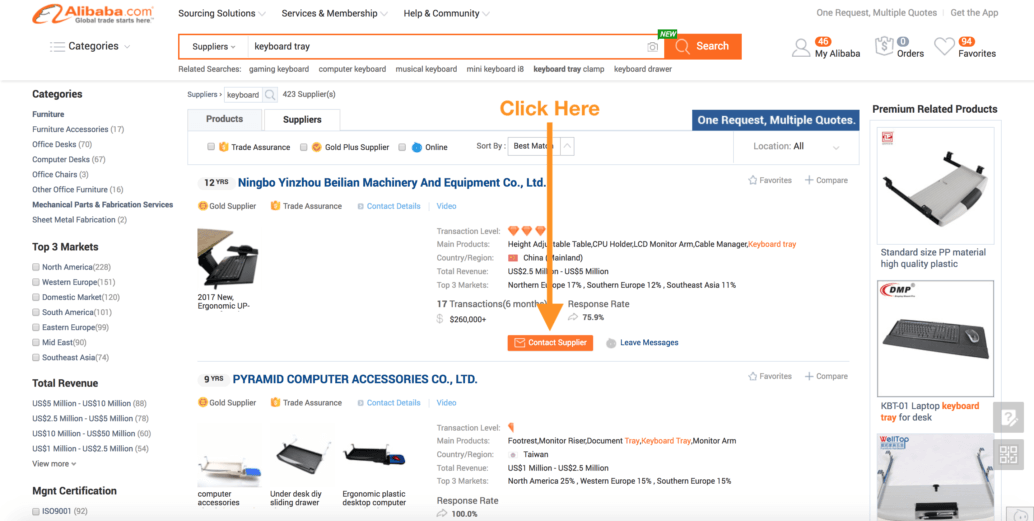The image depicts a comprehensive webpage layout from Alibaba.com, characterized by various navigational elements and product listings. At the top of the page, an orange Alibaba.com logo is prominently displayed. To the right of the logo, several drop-down menus labeled 'Sourcing Solutions,' 'Services and Membership,' 'Help,' and 'Community' are available for easy access.

Beneath the logo, another drop-down menu labeled 'Categories' is positioned towards the left. Adjacent to this, a horizontally extended search bar features its own drop-down menu, currently showing 'Suppliers' as the selected option. Within the search bar, the phrase 'Keyboard Tray' is entered, indicating a search query. Further to the right, icons for 'My Alibaba,' 'Orders,' and 'Favorites' allow users to manage their account and preferences.

On the left section of the page, the 'Categories' menu lists various product categories, providing users with a streamlined browsing experience. Following this, sections labeled 'Top 3 Markets,' 'Total Revenue,' and 'MG&T Certification' offer additional filters and insights into market performance and compliance standards.

To the right, the main content area displays several product images, particularly focusing on computer accessories. Each product is accompanied by detailed descriptions and pricing information, catering to prospective buyers seeking specific items on the platform.